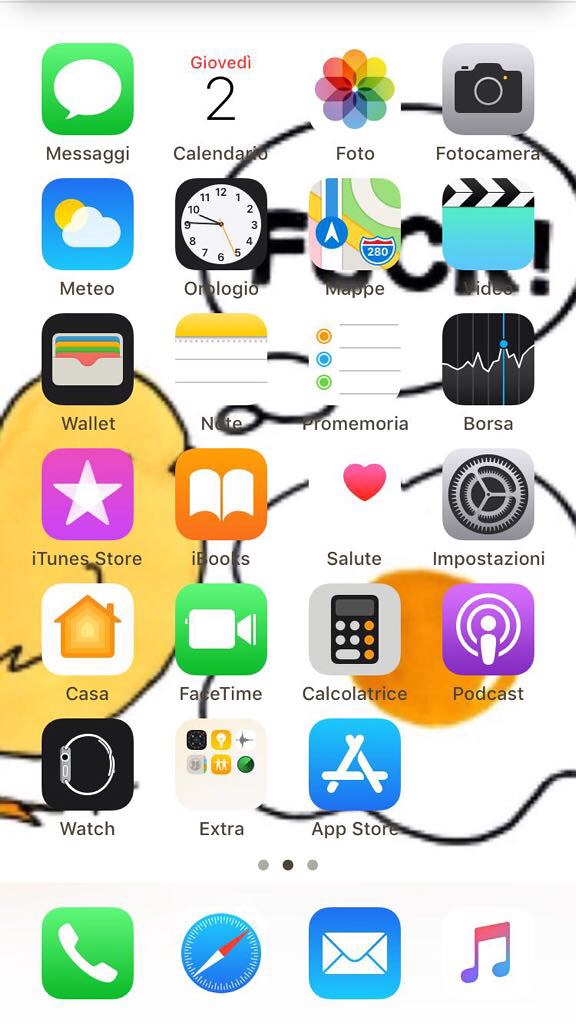The smartphone home screen is a vivid and crowded display, showcasing a colorful background with a distinct and humorous image. On the left, there's an outline of a small, yellow baby chick with a wing and a tiny foot sticking out. The chick has a thought bubble containing the word "F***!" in all caps, highlighting its frustration. Beside the chick, there's a quirky drawing of a fried egg with a wavy black outline and a bright yellow yolk, hinting at why the chick is unhappy.

The home screen features a typical grid layout with six rows of apps. Each row generally contains four apps, with the exception of the last row, which has three. The apps are labeled in Italian, suggesting the user's background or language preference:

1. **First Row:**
   - Mesaggi (Messaging app)
   - Calendario (Calendar)
   - Foto (Photos, with a rainbow-colored flower petal icon)
   - Fotocamera (Camera, with a basic black camera logo)

2. **Second Row:**
   - Meteo (Weather)
   - Orologio (Clock, with a clock face icon)
   - Mappe (Maps, reminiscent of the Google Maps icon)
   - Video (Featuring a black and white clapboard and a blue bottom screen)

3. **Third Row:**
   - Wallet (Depicted with interior slots for credit cards)
   - An unknown app obscured by the thought bubble
   - ProMemoria (Memo app, with a stack of three circular dots and lines for notes)
   - Borsa (Stock or finance app, indicated by a graph icon)

4. **Fourth Row:**
   - iTunes Store (Purple with a white star icon)
   - iBooks (Orange with an open book logo)
   - Salute (Health, with a red heart logo)
   - Impostazioni (Settings, with a gear icon)

5. **Fifth Row:**
   - Casa (Home, with a house logo)
   - FaceTime (Video call app, with a movie camera logo on a green background)
   - Calculatrice (Calculator, with a standard calculator icon)
   - Podcast (With a microphone icon on a purple background)

6. **Sixth Row:**
   - Watch (With an image of a smartwatch, resembling handcuffs)
   - Extra (A folder containing various apps)
   - App Store (With a stylized "A" made of three overlapping popsicle sticks)

Along the bottom of the screen are four standard icons:
- Phone
- Location
- Messaging
- Music

The busy and colorful home screen showcases a blend of functionality with a touch of humor, reflecting the personality and preferences of its user.